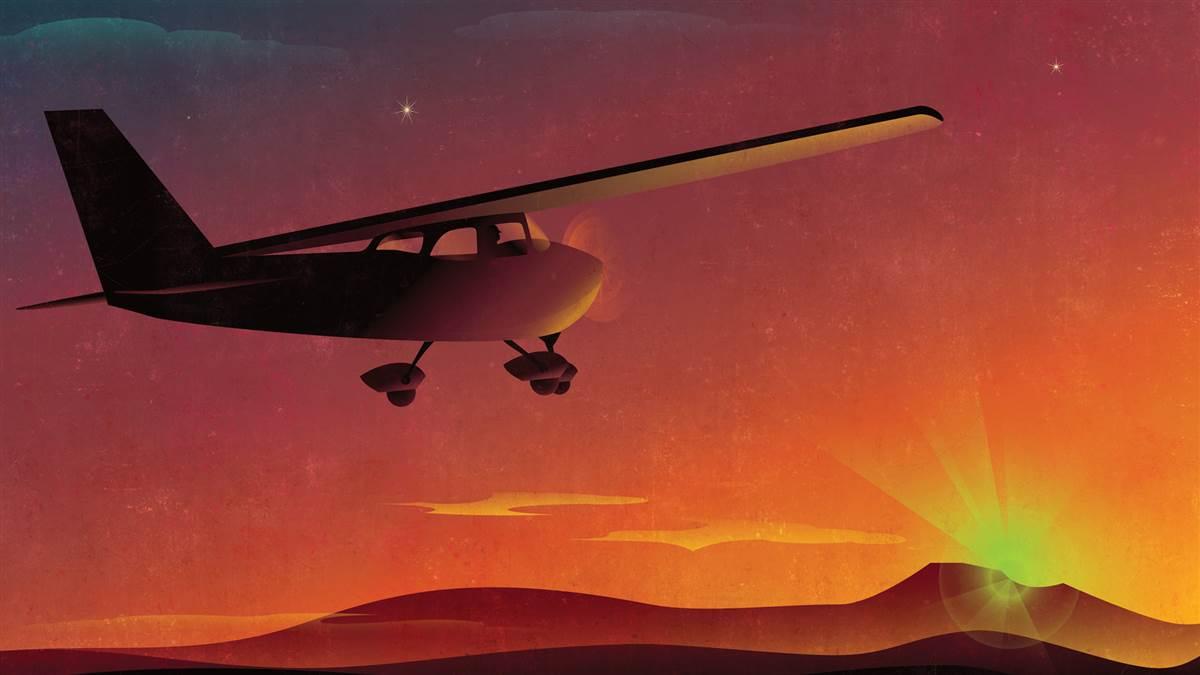This vector illustration showcases a minimalist yet detailed scene of a small Cessna propeller plane flying towards a vibrant sunrise or sunset. The plane, which appears to be a simple, old-fashioned design possibly accommodating one to four passengers, is centrally placed towards the left of the image. Its bottom wings are bathed in a yellowish hue from the sun, with motion-blurred propellers and black tail fins. The sky transitions dramatically from a glowing neon green sun close to the horizon, through shades of orange and red, to a dark gray in the top left corner, creating a striking gradient. Light wispy clouds float near the silhouetted mountain peaks at the bottom, enhancing the depth and atmosphere of the scene. Speckled stars in the sky add a whimsical touch to the artwork, while the textured patterns in the background suggest it might be an old print or a risograph, lending an antique feel to this beautiful illustration.